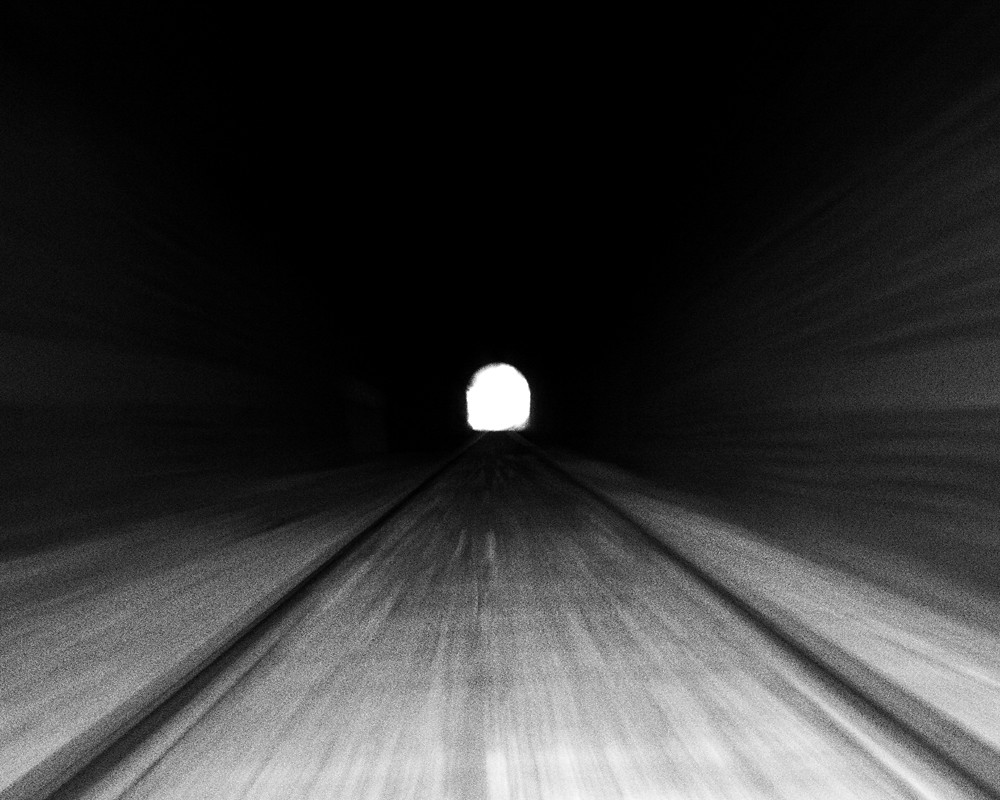This black and white photograph captures the perspective of a dark tunnel with a palpable sense of movement and mystery. The tunnel stretches ahead into a blend of shadow and light, characterized by a distinct white light at the far end, suggesting an exit or distant opening. The sides of the tunnel feature cement sidewalks or curbs, marked by black lines that emphasize their boundaries. The ground is gray, either lined with train tracks or cement tracks, contributing to the image's dynamic feel. The walls on both the left and right are also gray, blending into the blackness with a motion blur effect that heightens the sensation of traveling quickly through the tunnel. The overall composition exudes an artsy, almost surreal quality, drawing the viewer's eye towards the light at the end and evoking a feeling of rapid movement through this enigmatic space.